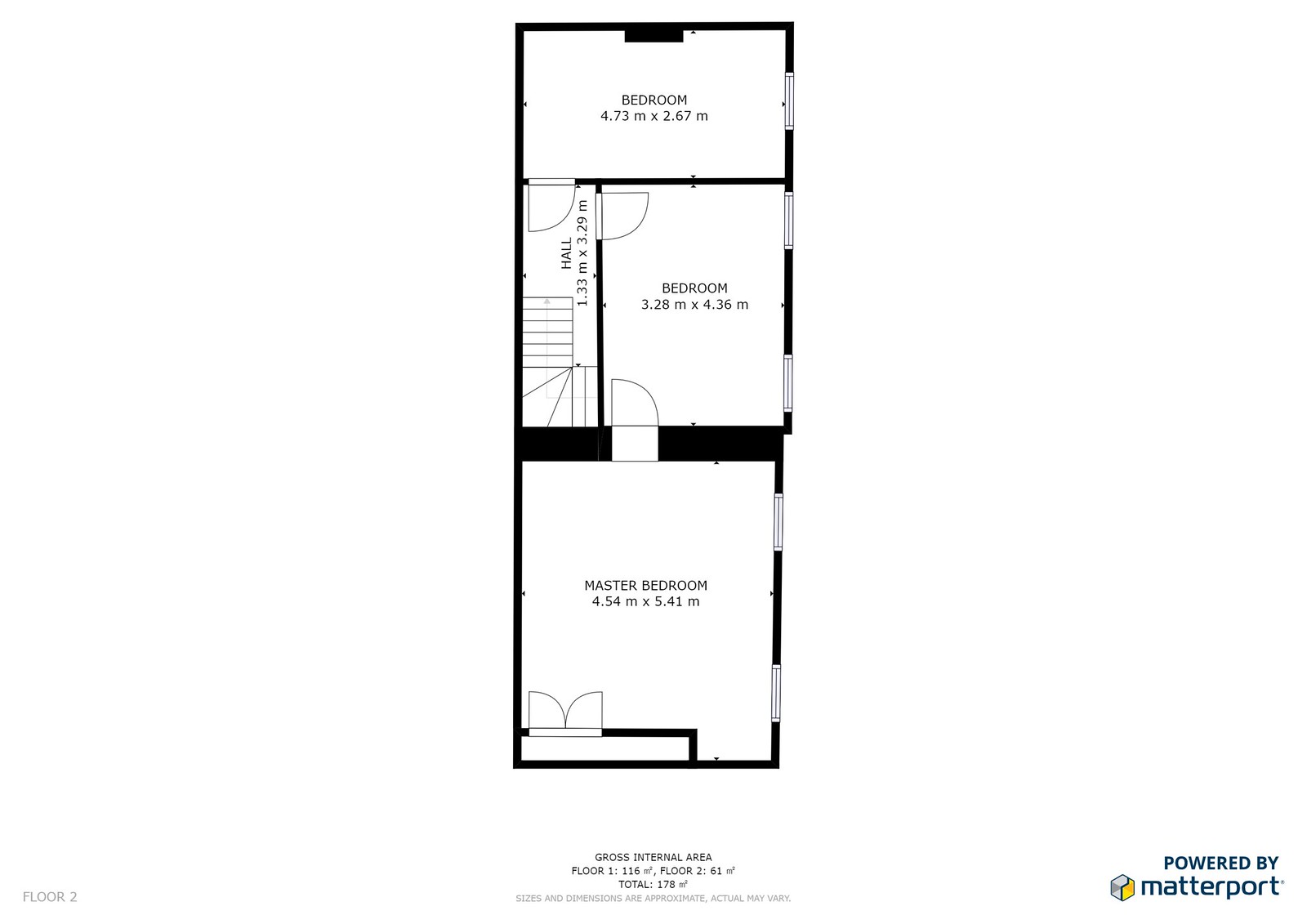This detailed digital blueprint mock-up showcases part of a house or apartment. The image features a vertically oriented, rectangular blueprint on the left, with a blank white background occupying the right half, save for the bottom-right corner, which hosts the black text "powered by Matterport" along with a six-sided geometric icon displaying a yin-yang pattern in gray and yellow to the left of the text.

The blueprint details three bedrooms, their dimensions, and surrounding architectural features. The topmost room is labeled "Bedroom" and measures 4.73 meters by 2.67 meters. Directly below it is another "Bedroom," occupying the right two-thirds of the midsection, measuring 3.28 meters by 4.36 meters. The left side of this section is designated as a hallway and staircase. The lower section features a "Master Bedroom" measuring 4.54 meters by 5.41 meters, equipped with a closet situated in the lower-left corner.

In addition, five windows are indicated as white gaps along the right wall of the blueprint. Below the diagram, additional text states the "Gross International Area," detailing the floor sizes: Floor 1 at 116 square feet and Floor 2 at 61 square feet, making for a total of 178 square feet.